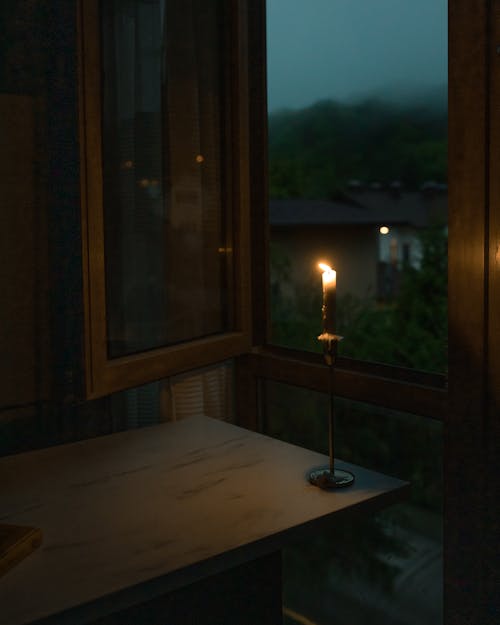This image is a detailed color photograph in portrait orientation, capturing the serenity of an interior lit by a single candle during nighttime or dusk. The lit candle is positioned slightly to the right of center, resting on a rectangular, light brown wooden table near the bottom of the frame. It is held by a tall, metal candlestick with a dark finish. The candle's flame flickers inward, providing the only light source in the room and accentuating the shadows on the dark surrounding wood paneling. 

Directly behind the candle is an open, vertical window with brown wooden frames swung inward, revealing an outdoor landscape. The view through the window showcases a mist-covered hill descending into another hill, partially obscured by a shroud of gray-white fog. The sky outside is a hazy dark bluish-gray, adding to the moody atmosphere. In the distance, the roof of another home peeks through the foliage of trees and bushes, bringing a sense of depth to the scene. The overall composition of the photograph exemplifies photographic representational realism, emphasizing the interplay of light and shadow in this quiet, contemplative moment.